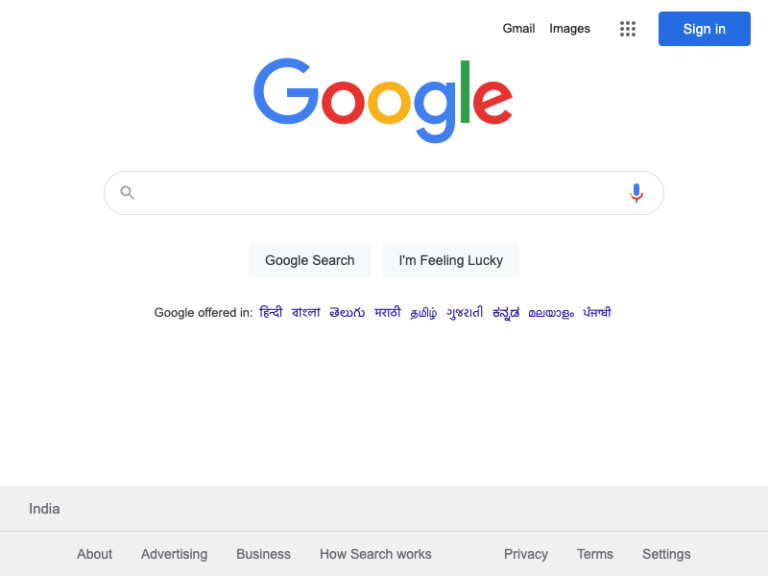In this image, the main focal point is a Google homepage. Prominently featured at the top-center is the iconic Google logo, displayed in its signature color pattern of blue, red, yellow, blue, green, and red. At the top-right corner of the page, there are quick access links labeled "Gmail," "Images," and a "Sign In" button. Below these links is the central search field, which includes a search bar, a magnifying glass icon for initiating searches, and a microphone icon for voice input. 

Beneath the search bar, there are two buttons: "Google Search" and "I'm Feeling Lucky." Under these buttons, a language selection option is displayed with nine different languages listed—all excluding English. At the bottom of the page, a footer area provides links to various Google services and information, including "India," "About," "Advertising," "Business," "How Search Works," "Privacy," "Terms," and "Settings." The page design maintains the characteristic minimalistic Google aesthetic.